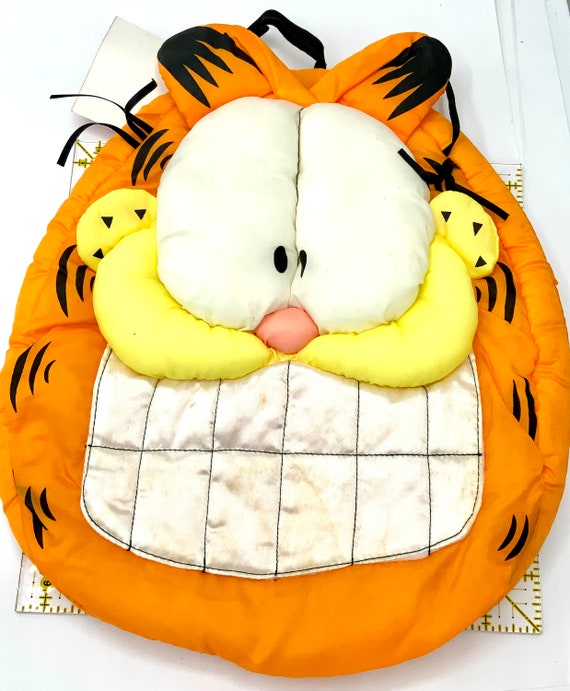This photograph depicts a large, homemade fabric representation of Garfield's head, set against a white background. The object, which resembles either a backpack or an unstuffed pillow, showcases Garfield's iconic features: a big, round orange face with black stripes, large, shiny white teeth, and big white eyes with tiny black pupils. His orange ears with black details stand out near the top of the piece. The face includes poofy details on the eyes and nose, and a yellow snout. The edges of the white background feature gold-trimmed corners poking out from underneath the Garfield head, while a black rope handle at the top and a white tag in the upper left corner add functional elements. The presence of an acrylic ruler in the background appears to indicate the dimensions of this arts and crafts project.